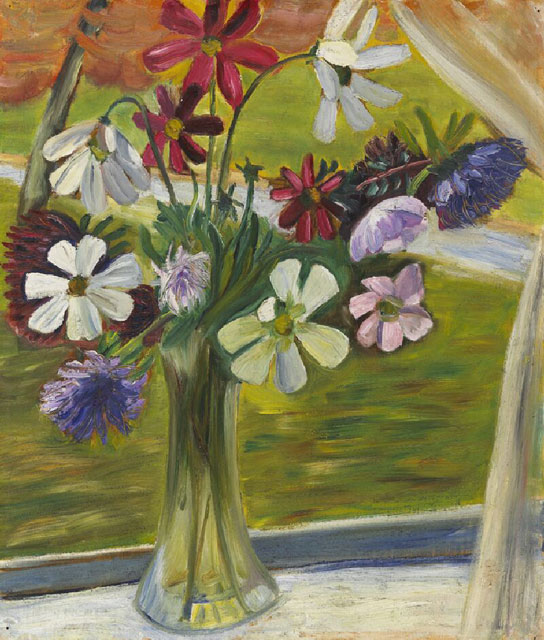The image is a detailed painting of a clear glass vase, narrow at the top and wider at the base, sitting on a narrow white windowsill. The vase is filled with a vibrant assortment of flowers, prominently featuring cosmos in hues ranging from white and pink to deep red and purple, some with yellow centers. Accompanying the cosmos are daisies and lilies, with lush green leaves interspersed among the blooms. On the right side of the image, a white curtain partially frames the scene. Outside the window, a green expanse of grass is visible, intersected by a narrow white path that adds depth and dimension to the painting. The brush strokes create a dynamic interplay of colors, particularly noticeable in the maroon-tinted red and the occasional greenish tinge to some of the petals. The composition suggests a serene and scenic view, possibly of someone's front yard.